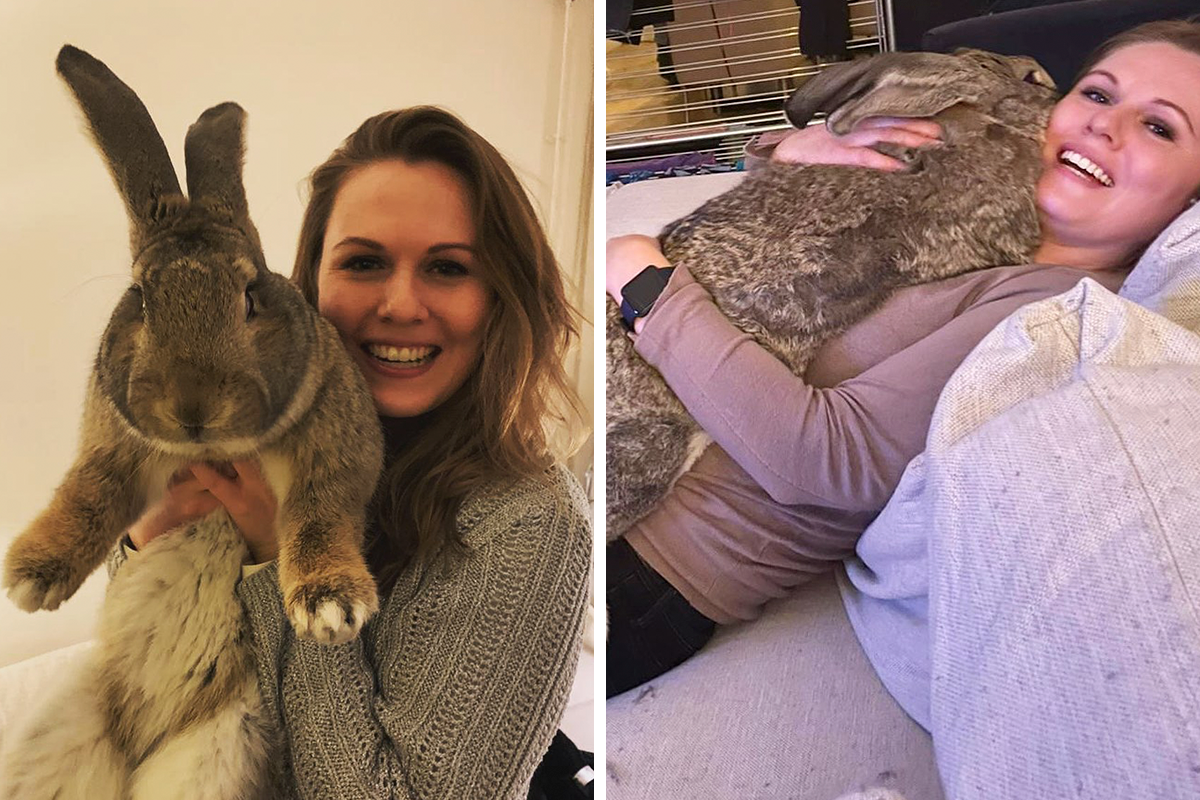The image is a split photograph featuring a woman with a very large rabbit, with a distinct white line dividing the two parts. In the left picture, the woman with auburn-colored hair is wearing a tan sweater with an ornate woven design on her left shoulder. She is holding an enormous, living rabbit upright with both hands. The rabbit has incredibly long ears that nearly match the length of her head, and his face is about the size of hers as well. His white belly is visible, along with his substantial legs and paws, which dangle well below her waist. The second picture on the right shows the same woman reclined on a couch over two white pillows, wearing a pinkish-gray shirt and an Apple watch. She appears to be hugging and nuzzling the rabbit, which stretches from her eye level down below her knees. This giant rabbit, with brown fur accented by white spots on his back and smooth white fur on his belly, looks almost as big as a small dog and provides a striking contrast in size to the woman.